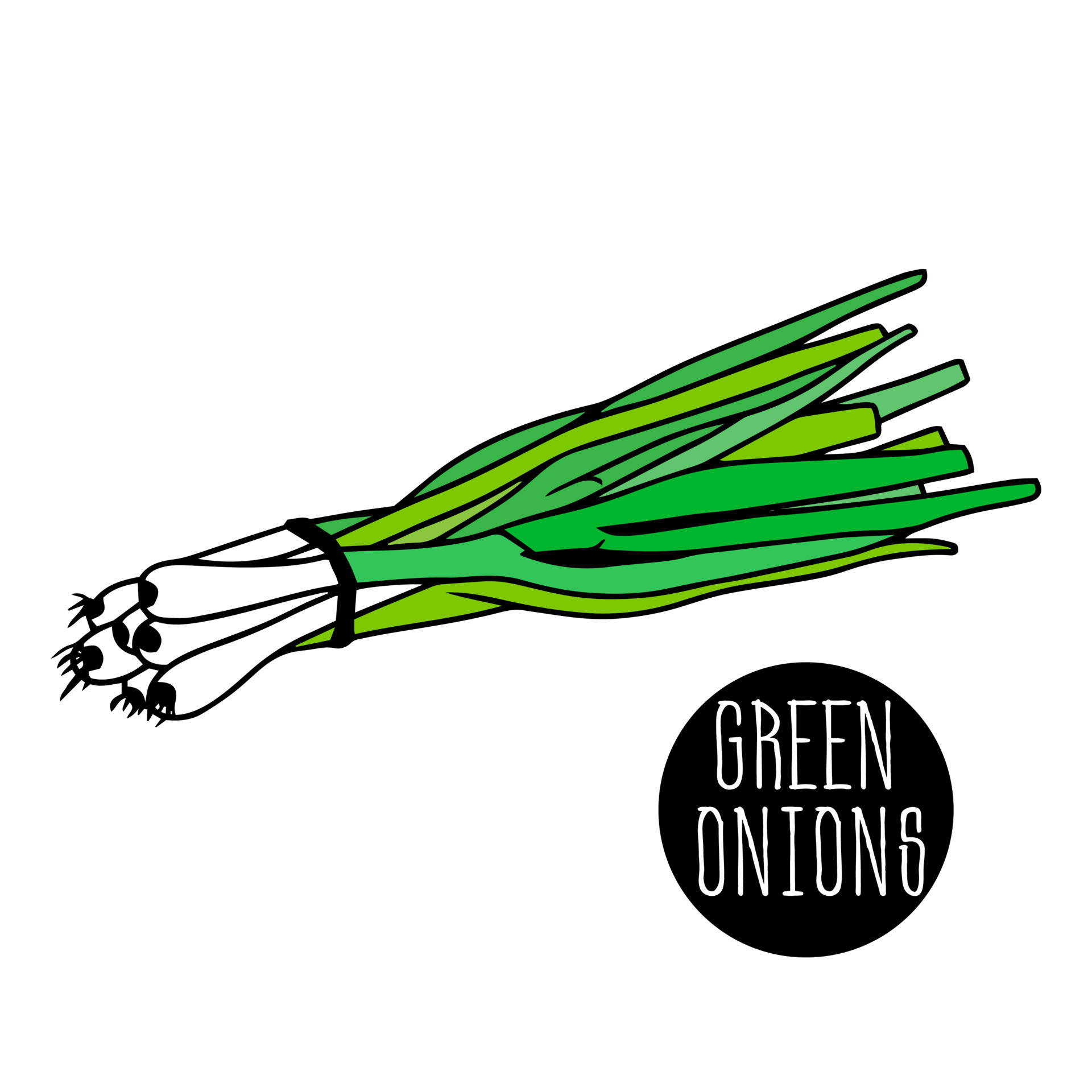This detailed drawing features seven green onions, also known as scallions, laid on their sides against a completely white background. The green onions are tied together with a black rubber band located about an inch or two above the white bulbs, where the stems transition from the round, white base to their vibrant green tops. The green stems showcase an array of colors, including electric green, medium green, and lighter green hues. The roots of the bulbs are depicted in black. In the bottom right corner of the image, there is a black circle containing the words "green onions" written in white typeface. The composition suggests a bunch of green onions as they might appear ready for sale in a supermarket.